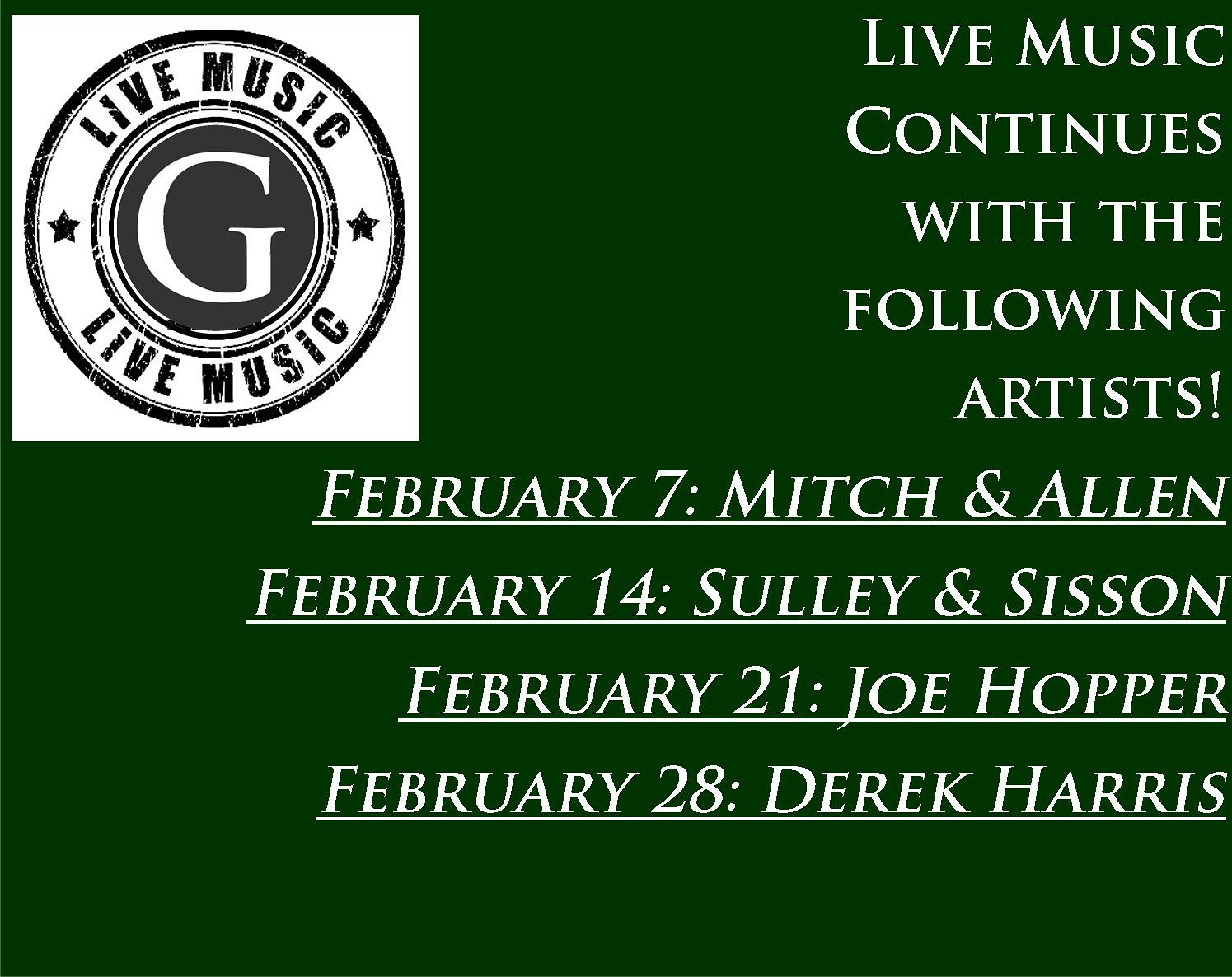The horizontally oriented image features a green background with white lettering. In the top left corner, there is a circular logo with the words "live music" encircling a large "G" in the center. Adjacent to this logo, the text in capital letters reads: "LIVE MUSIC CONTINUES WITH THE FOLLOWING ARTISTS." Below this heading are four lines, each listing a date followed by an artist or duo: "February 7th: Mitch and Alan," "February 14th: Sully and Sisun," "February 21st: Joe Hopper," and "February 28th: Derek Harris." The image resembles a postcard and likely indicates monthly updates about live music events.